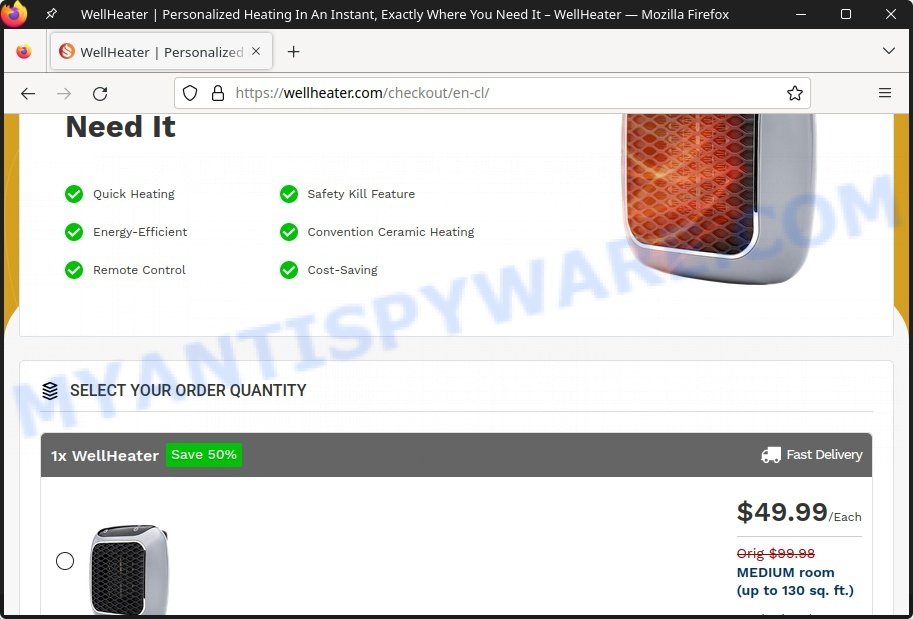This rectangular, horizontally-oriented screenshot prominently displays a promotional banner for the "Well Heater" product on a webpage. At the top, a black banner features the Mozilla Firefox icon in the upper left corner, followed by the text "Well Heater" in white. To the right, the slogan reads: "Personalized heating in an instant, exactly where you need it." Below the banner, a button labeled "Well Heater personalized" is visible.

In the main section of the image, set against a white background, there is a detailed presentation of the heater. On the right side, a color photograph showcases the device, which is silver with a brown interior. To the left of the photo, bold black text declares, "Need It." Below this headline, several features of the Well Heater are listed with green bullet points featuring white check marks: "Quick Heating," "Energy Efficient," "Remote Control," "Safety Kill Feature," "Convenient Ceramic Heating," and "Cost Saving." The price is marked in the lower right corner of the image as "$49.99 each."